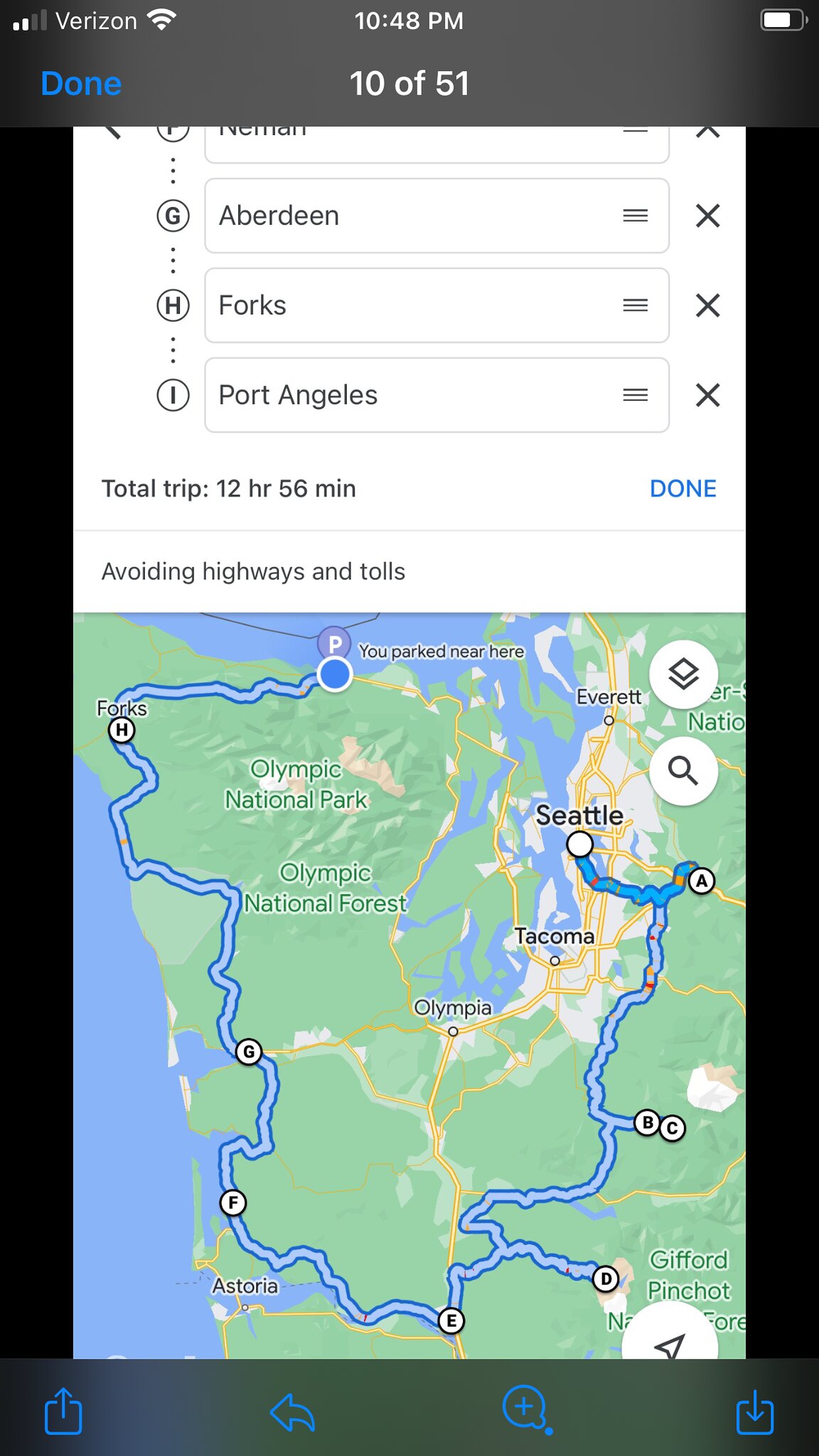The image is a detailed screenshot from a phone displaying a map app, providing directions for a multi-stop journey through Washington state. At the top of the screen, the status bar shows "Verizon" as the carrier, with a full Wi-Fi signal indicator, the time "10:48 PM," and a battery icon without a percentage. The top left corner also includes a blue "Done" button, and beneath the time, it reads "10 of 51." The main portion of the screen displays a route starting in Seattle and traveling through various points, including Neiman, Aberdeen, Forks, and Port Angeles, totaling a 12-hour and 56-minute trip while avoiding highways and tolls. The map itself is highlighted in green, indicating land, with a vivid blue path illustrating the journey across the state's western side.